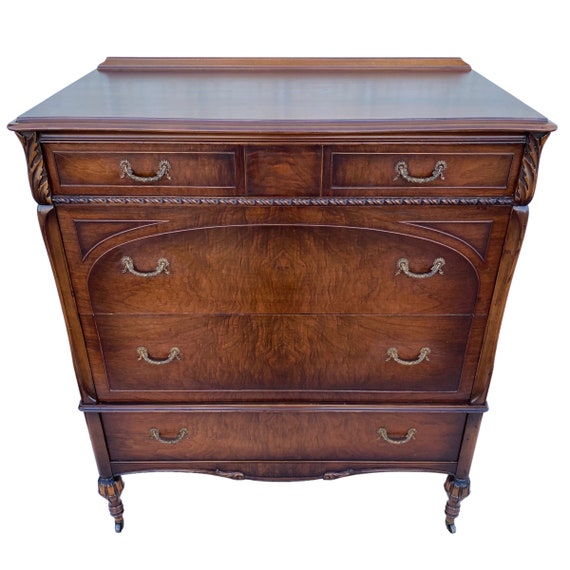This image depicts an antique wooden dresser with a rich, dark brown, possibly cherry finish. The dresser is characterized by its sleek and narrow front legs, which are supported by small, old-fashioned wheels. The front facade boasts a seamless grain pattern that runs vertically down its length. The piece comprises five drawers: three spacious drawers at the bottom and two narrower ones at the top. The bottom two levels of drawers are accentuated by a decorative border, while the corners and tops feature intricate adornments. Each drawer is fitted with drop-down loop handles, arranged symmetrically. The top surface of the dresser is flat and shiny, reflecting its top-notch condition, and a thin piece of wood rises slightly at the back of this surface. At the very bottom, a small decorative panel garnishes the base, completing the elegant and timeless design.